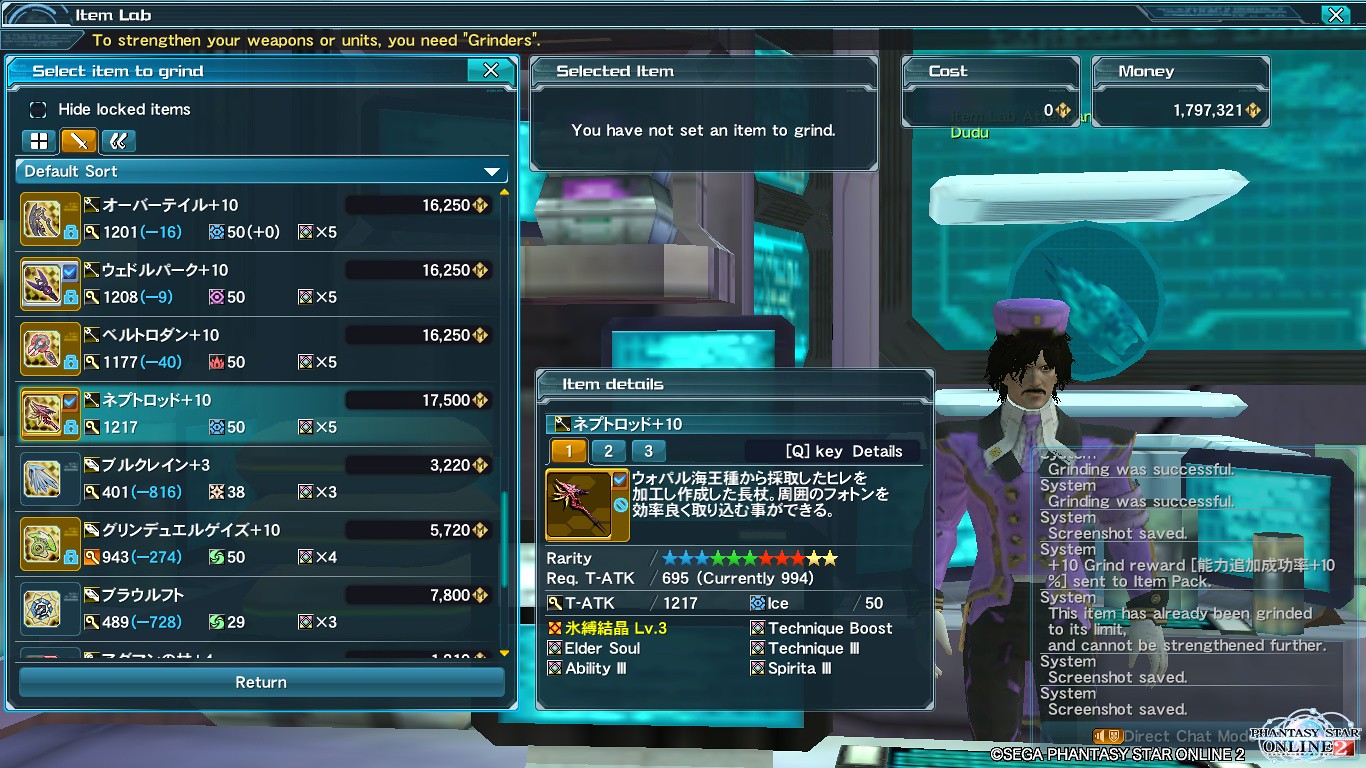This detailed screenshot captures a moment from the video game "Phantasy Star Online," developed by SEGA. The interface is predominantly blue and green, with several menus and a control panel displayed prominently. The text mainly consists of Japanese characters, although there are notable English phrases such as "select item to grind," "select item," "money cost," "item details," and "key details." 

To the right side of the screen, a character resembling a custom-made avatar stands out. This character, dressed in a distinctive purple bellboy or butler suit, has a black mustache and hair reminiscent of Michael Jackson's style. The setting appears slightly futuristic, with a mainframe-like background suggesting advanced technology. The interface includes options related to strengthening weapons or units using grinders, and other text indicating system messages, rewards, and a saved screenshot. Overall, the visual style and elements suggest the game has a nostalgic design, evoking early 2000s aesthetics.